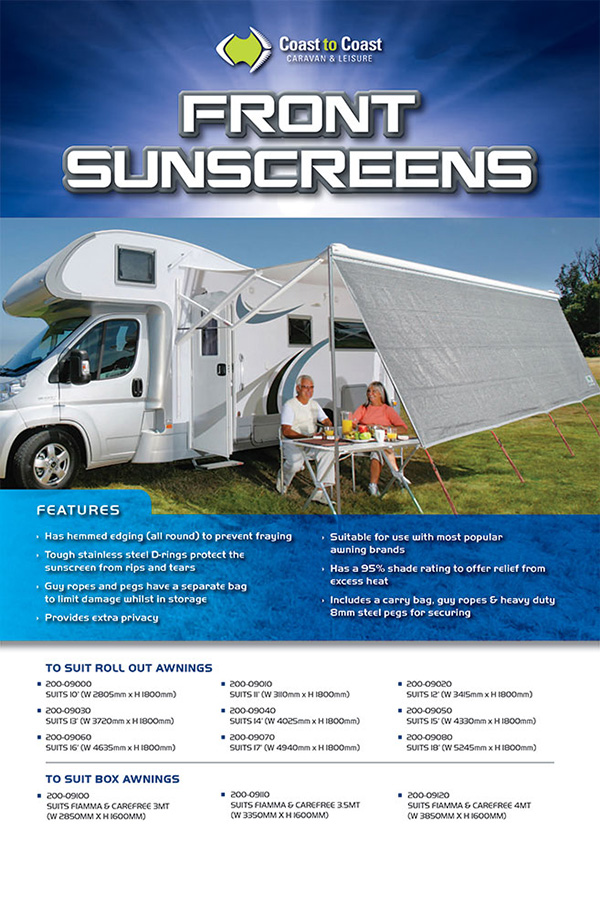The image is an informational flyer for a product by Coast to Coast Caravan and Leisure, prominently displaying their Front Sunscreen for RVs. The layout features a large central image of a white RV with a black and blue-gray swooping decal, parked on green grass under a blue sky. The RV is positioned to the left side of the image, with windows above and below the decal line. Extending from the RV is an awning, under which a couple—a man in a white t-shirt and a woman in a pink outfit—are seated at a table, enjoying a meal in the shade provided by the sunscreen. 

The text on the flyer provides detailed product features: "Front Sunscreen" in bold, white bubble letters on a blue background, followed by a list of benefits including hemmed edging to prevent fraying, tough stainless steel D-rings for durability, guy ropes and pegs with separate storage to limit damage, and 95% shade rating for heat relief. The product also includes a carry bag, guy ropes, and heavy-duty 8mm steel pegs for securing the sunscreen. Additionally, smaller blue text mentions compatibility with roll-out and box awnings. The image and text collectively convey a practical, user-friendly product designed to enhance leisure and comfort during RV outings.